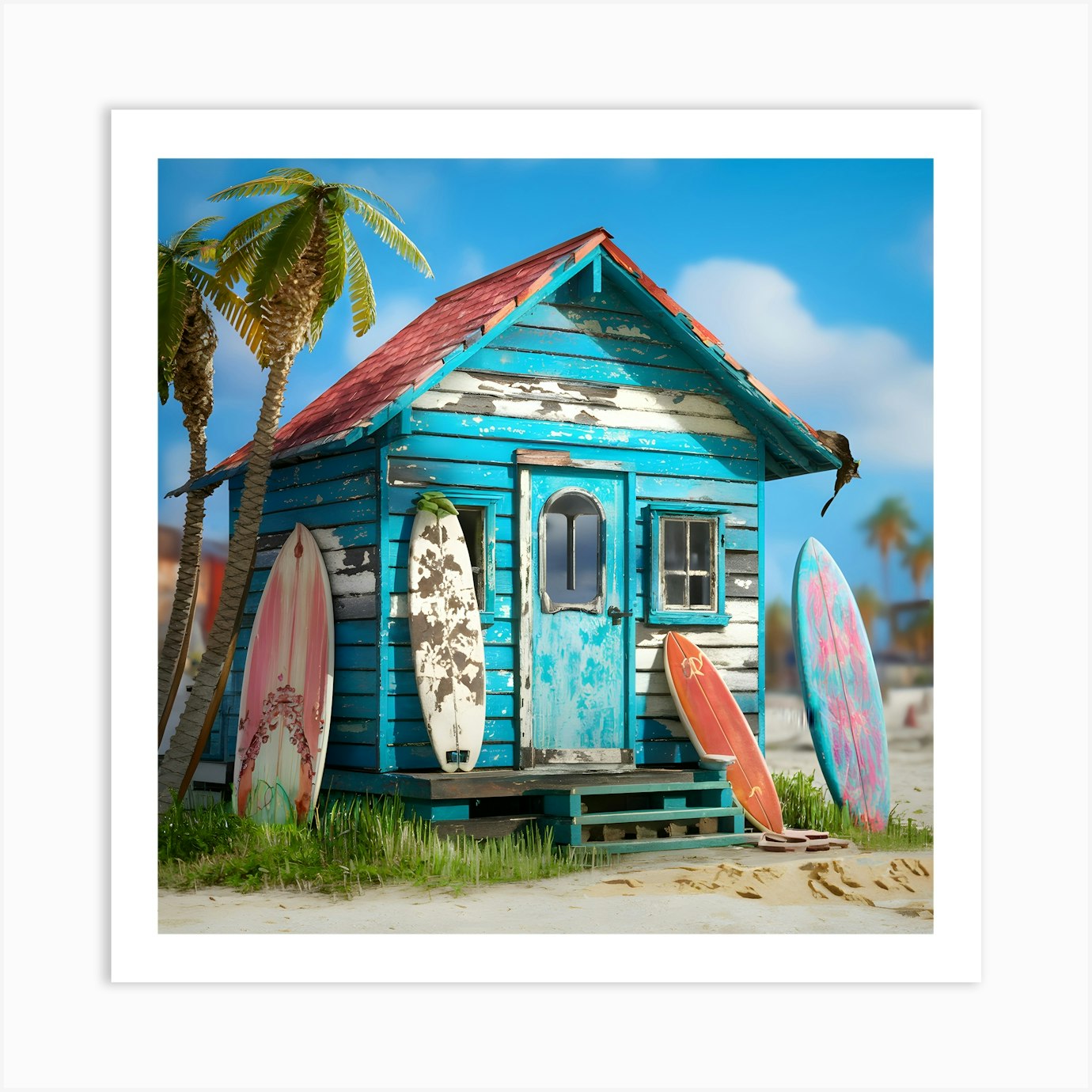The image is a vibrant and colorful digital illustration framed with a clean white border, resembling a Polaroid picture. It portrays a dilapidated tropical beach hut, about 50 square feet in size, with peeling turquoise clapboard walls revealing layers of white and gray underneath. The roof is made of reddish shingles that appear to be worn and peeling. The hut features a door with an arched glass window and two small four-pane windows flanking the door, with a tiny porch accessible via two or three steps.

To the left of the hut, two palm trees lean slightly towards the roof, adding a tropical atmosphere. Surrounding the base of the hut are patches of green beach grass transitioning into sand, which extends into the background where more sand and blurred palm trees can be seen, under a bright blue sky with fluffy white clouds.

Leaning against the hut are three surfboards of various designs: a small red surfboard with a monogram 'P' under the right window, a broad pink and white surfboard covering almost the entire left window, and a white surfboard leaning on the left side of the hut. Further right, stuck upright in the sand, is a blue surfboard adorned with pink palm trees.

This striking illustration captures the essence of a serene, somewhat nostalgic tropical beach scene dominated by the old, yet colorful and personality-filled surfer shack.